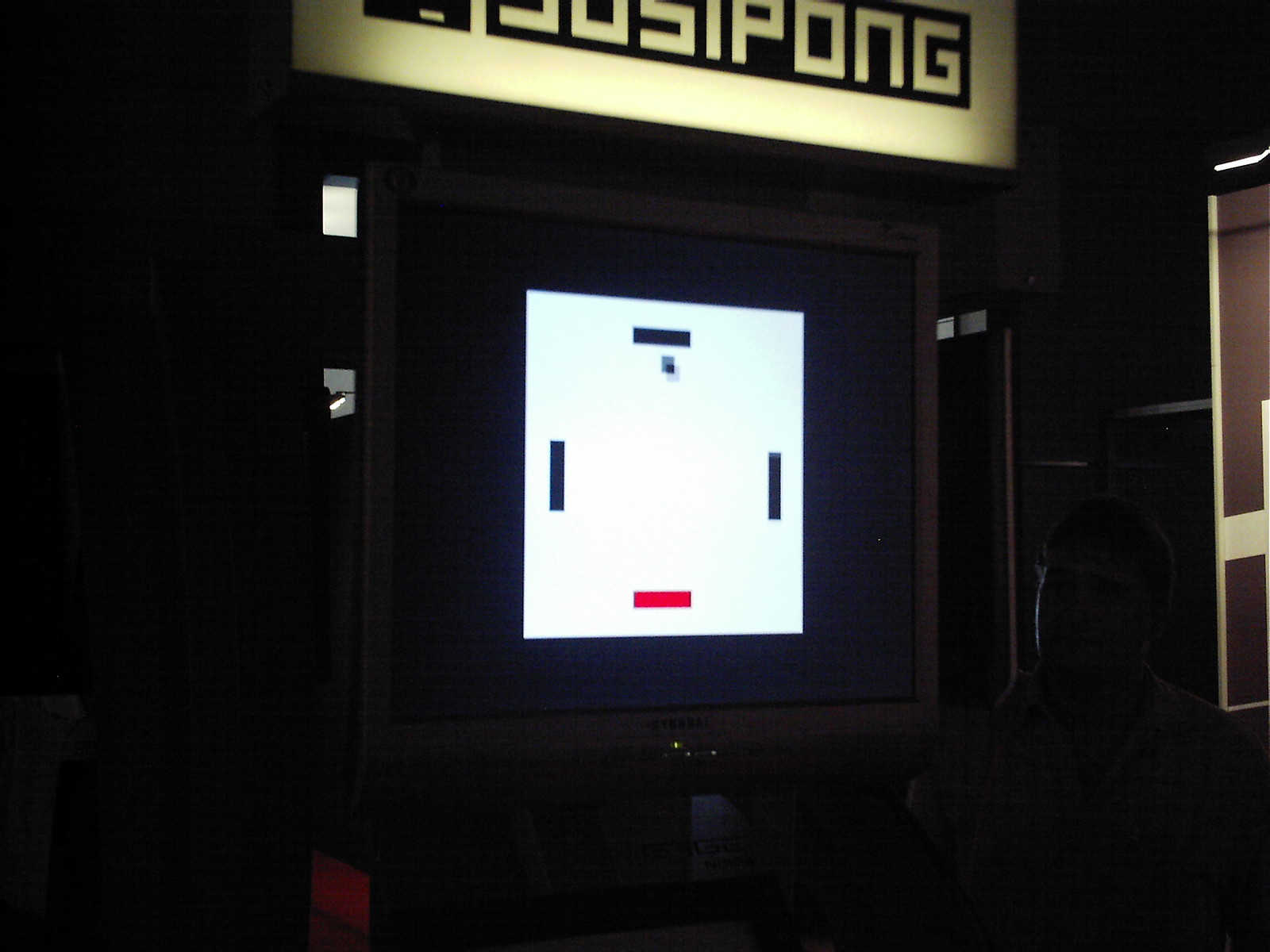This is a somewhat dark photograph of an old-style video game console, displaying what appears to be the game Pong. The background of the image is almost entirely black, adding to the low-quality, pixelated appearance of the scene. A large, partially legible sign is perched atop the console, the discernible portion of which reads "PONG," preceded by indistinct characters. 

The console's screen is prominently featured in the center of the photo. The display consists of a dark blue background housing a white square area, within which appear three black lines—one at the top and one on each side—along with one red line at the bottom. In the center is a small square that seems integral to the game being played, possibly Pong.

To the lower right side of the console, faintly visible in the shadows, is a young man. His body faces towards the left, though his head tilts slightly to the right, gazing intently at the screen. Off to the right of the console, there is a small, gold-lined display window with a black interior.

This intriguing, nostalgic scene captures a moment of interaction with classic video gaming, enveloped in the mystery and ambiance of a dimly lit setting.